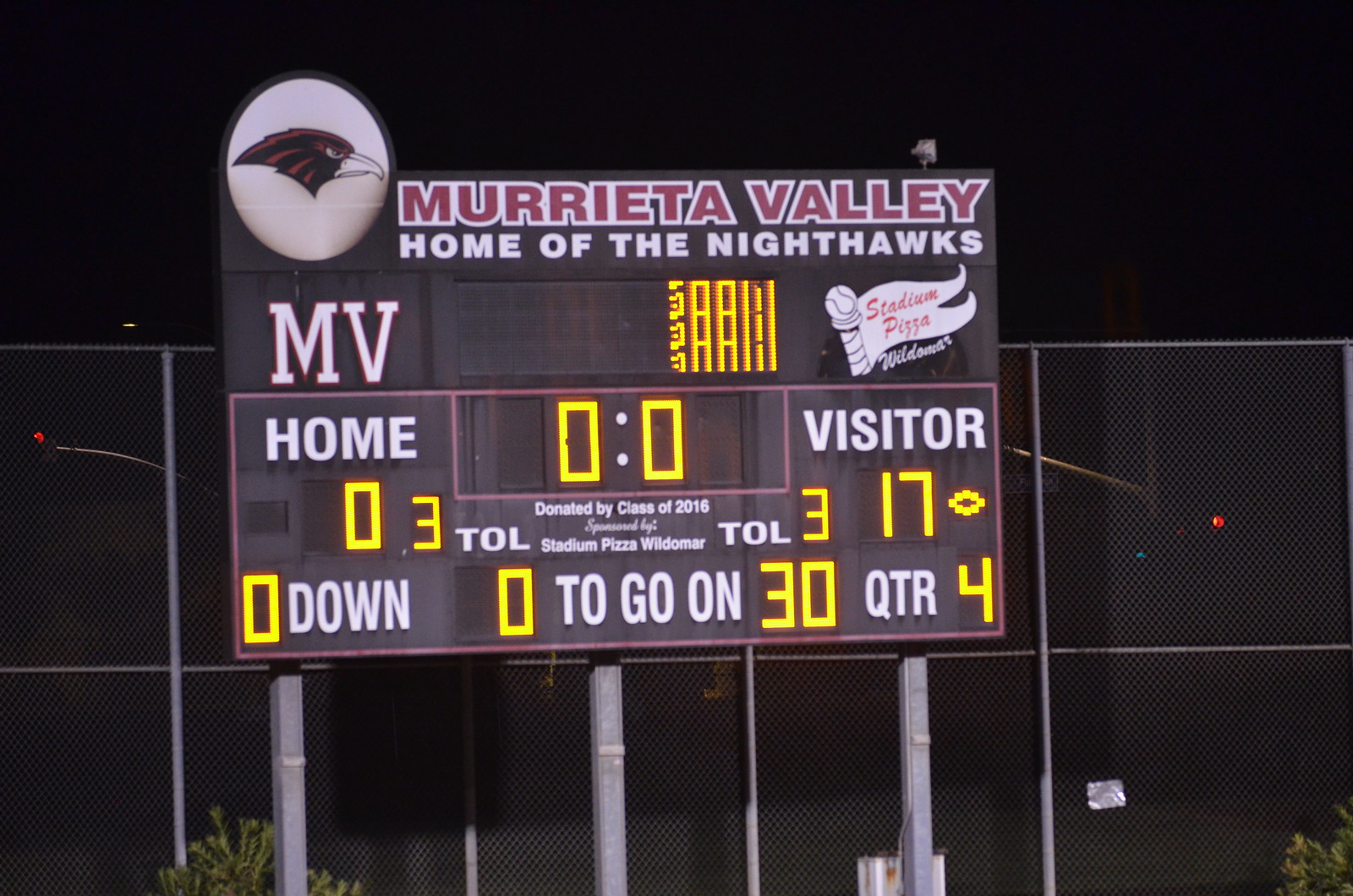The image depicts a prominently illuminated high school sports scoreboard situated against a steel mesh fence in an outdoor ballpark during the evening. The scoreboard, belonging to Marietta Valley High School, proudly displays the team name "Marietta Valley, Home of the Nighthawks" with a logo of a Nighthawk's head inside a white circle. The colors on the scoreboard are primarily red and black, reflecting the school’s mascot colors. Below this header, the scoreboard shows the home team "MV" with a score of 0 versus the visitor team's score of 17. The game is in the fourth quarter, with other indicators showing '0 down', '0 to go', and '30' remaining in the period. The time displayed is 00:00, with a total of 3 for the timeout under both teams. A small advertisement for "Stadium Pizza" is visible in the upper right corner. Additionally, a message underneath the central time display reads "donated by class of 2016." The background features a double-tier high steel mesh fence, suggesting the game takes place in a well-contained field.